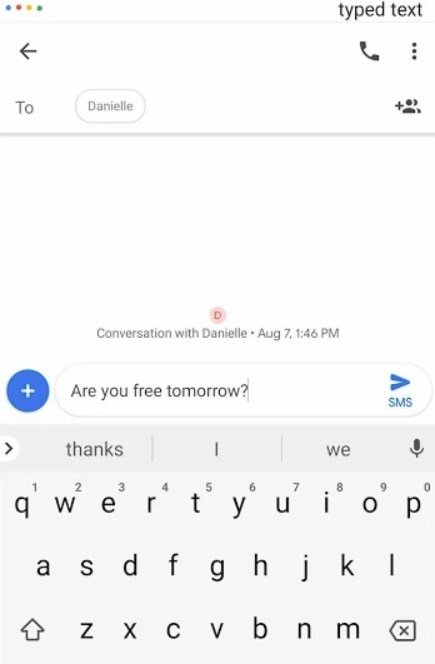In this image, we see a screenshot of a messaging app interface on a mobile device. The top-left corner features four small dots in blue, red, yellow, and green, suggesting a recognizable app color scheme. On the right-hand side at the top, the words "typed text" are visible, indicating the field for composing messages.

Below this section, the interface includes a back arrow, a phone symbol, and a three-dot menu icon for options or settings. The header of the conversation indicates it is addressed "To: Danielle," accompanied by a small plus icon near a people image, allowing the addition of more recipients.

The main part of the screen is a blank area where the conversation history would appear. At the bottom of this blank area is a red circle with the letter "D" inside it, and the text "Conversation with Danielle, August 7, 1:46 PM."

Further down, we encounter a user input area featuring a round blue button with a plus sign. Adjacent to it is a text entry box containing the message "Are you free tomorrow?" To the right of this message, there is a small blue arrow pointing right, and beneath this arrow, the word "SMS" is displayed.

Finally, at the bottom of the screen is the mobile device keyboard. The top row displays suggested words such as "thanks," "I," and "we," and there is also a microphone icon for voice input. Below this row are the standard keys of a mobile keyboard.

This detailed description captures the layout and elements of the messaging app interface as depicted in the screenshot.